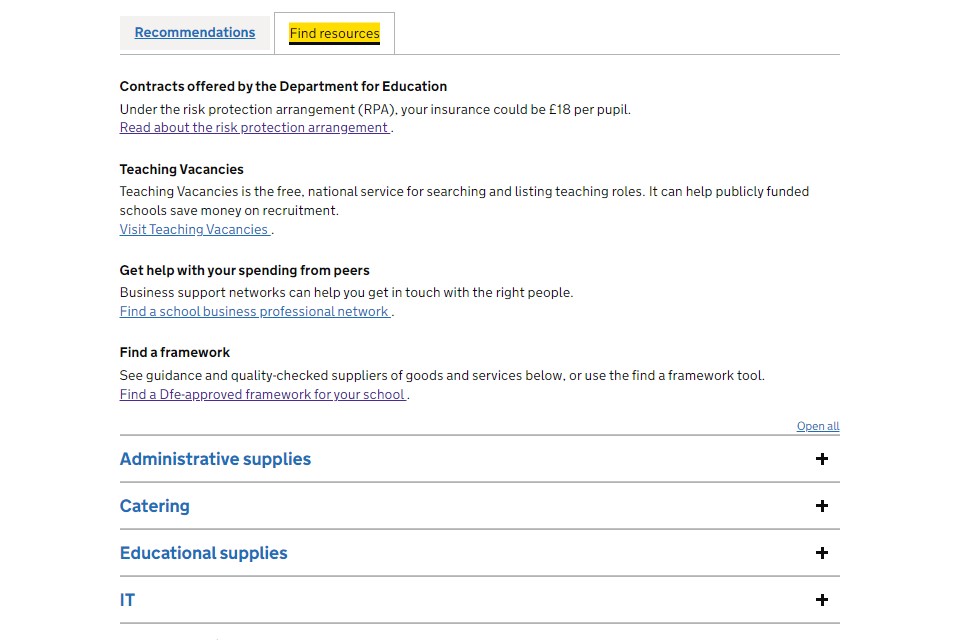Here's a detailed and cleaned-up descriptive caption for the image:

---

The interface features two top tabs: one titled "Recommendations," which is blue and underlined, and another labeled "Find Resources," highlighted in yellow with a black underline. Below these tabs, a section header reads, "Contracts offered by the Department of Education." Further down, the text explains the Risk Protection Arrangement (RPA) insurance, noting, "Under the Risk Protection Arrangement (RPA), your insurance could be £18 per pupil." There is a hyperlink labeled "Find the Risk Protection Arrangement" displayed in purple and underlined.

Another section details "Teaching Vacancies," describing it as, "Teaching Vacancies is the free national service for searching and listing teaching roles. It can help publicly funded schools save money on recruitment." A call-to-action, "Visit Teaching Vacancies," is in blue and underlined.

Further down, another section reads, "Get help with your spending from peers. Business support networks can help you get in touch with the right people. Find a school business professional network," also in blue and underlined.

The next section highlights using frameworks: "Find a framework. See guidance and quality check suppliers of goods and services below, or use the find a framework tool. Find a DFE-approved framework for your school," underlined in purple.

At the bottom, categories such as "Administrative Supplies," "Catering," "Educational Supplies," and "IT" are listed in blue with grey lines separating them. Each category ends with a plus sign (+) on the right side. Additionally, there is an "Open All" option positioned at the top right of these categories.

---